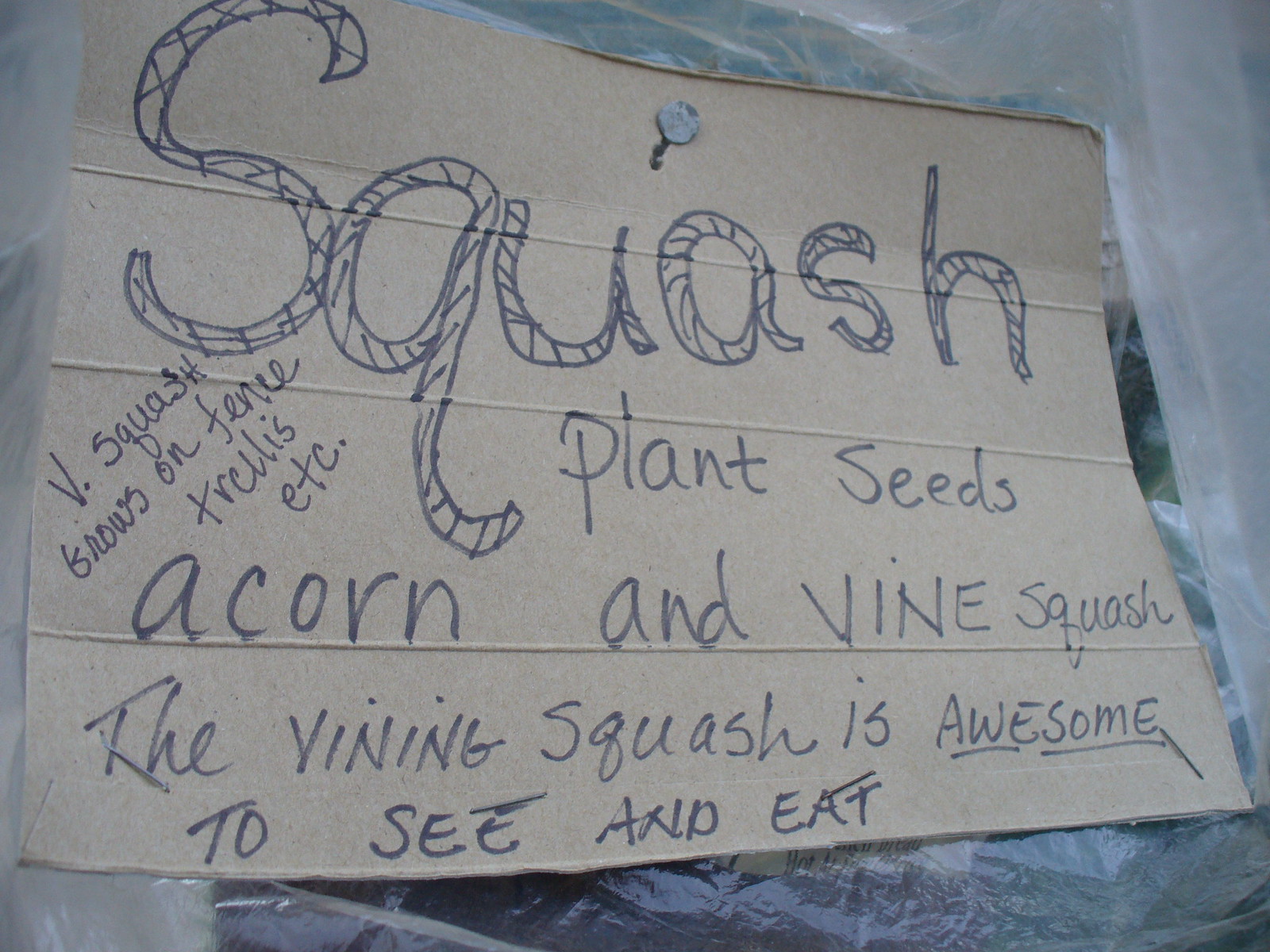A cardboard sign tacked to a glossy, possibly plastic surface with a nail through the top displays an enthusiastic message about squashes. The top of the sign features the word "squash" in large, outlined letters filled with zigzag lines for emphasis. Beneath this, written diagonally on the left side, it reads "V-squash grows on fence, trellis, etc." Further down, it instructs readers to "plant seeds" and lists "acorn and vine squash." At the bottom of the sign, a note celebrates the plants: "The vining squash is awesome," with "awesome" doubly underlined for effect. The final line proudly states, "to see and eat."